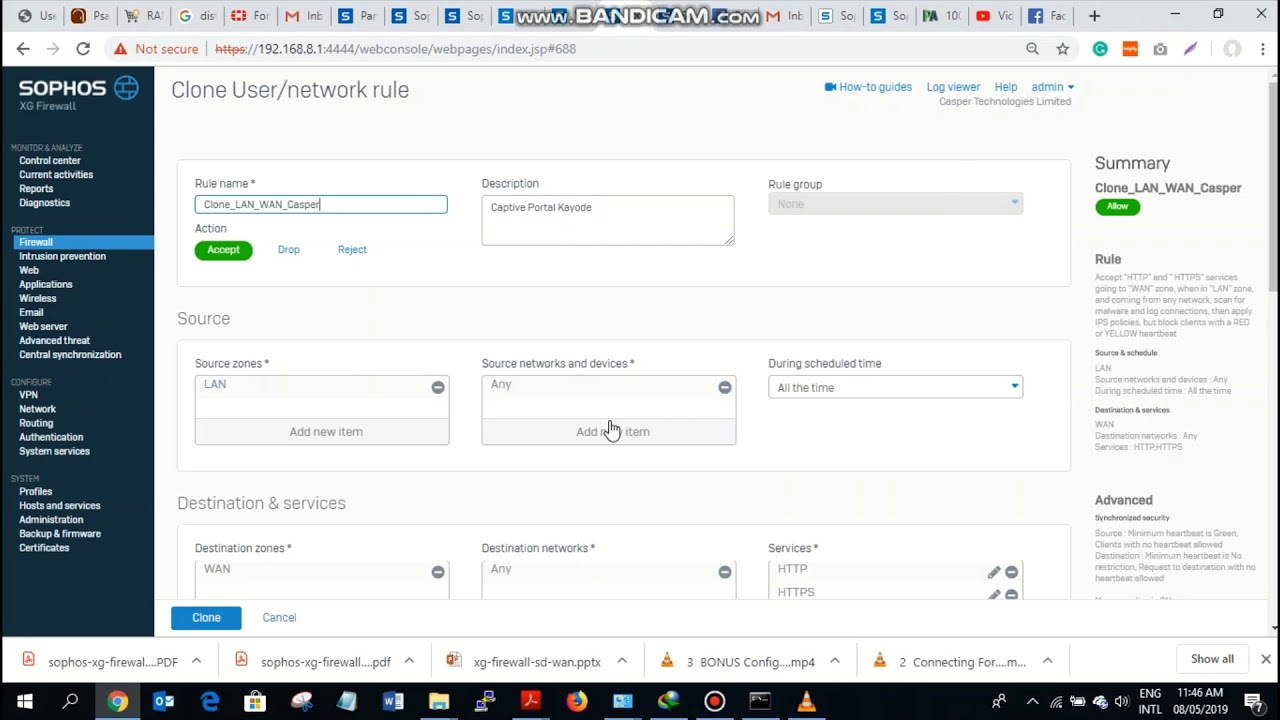The image is a screenshot from a website page belonging to Sophos, spelled S-O-P-H-O-S. The page features a navigational sidebar on the left, which includes various clickable items that direct users to different sections of the site. The main content area of the page is displayed in a yellowish-tan background and is centered around a form labeled "Clone User/Network Rule."

The form comprises several white fields organized into rectangular sections. At the top is a field labeled "Rule Name," followed by two more fields labeled "Description" and "Rule Group." Below these fields is a green "Accept" button. Further down, there are sections labeled "Source" and "Destination and Services." 

The "Source" section includes fields for "Source Zones," "Source Network and Device," and "During Scheduled Time." The "Destination and Services" section has fields for "Destination Zones," "Destination Networks," and "Services," with options for "HTTP" and "HTTPS" specified under the "Services" field.

At the bottom left of the form is a blue button labeled "Clone." Additionally, the bottom area of the page contains an assortment of clickable icons and a "Show All" button.